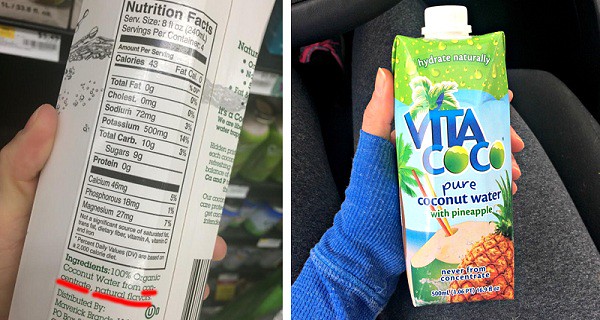The image consists of two side-by-side photographs, each depicting a paper-based coconut water container held by a Caucasian individual. 

On the left, the background features blurred shelves of cans in a grocery store's refrigerated section. The container itself displays nutritional facts printed in black on a white rectangle with bold black lines. Key details of the label include serving size information, cholesterol content, and some words underlined in red. The bottle is held by a person whose thumb and the tips of their index and middle fingers are visible.

On the right, a woman dressed in a long-sleeved blue thermal shirt holds a rectangular Vita Cocoa bottle with her left hand, exposing her left thumb and inner palm. The bottle features a white cap, a green top section, and light blue lower section. The front design showcases an ocean or beach view with a cut coconut and pineapple, alongside the brand name "Vita Cocoa" in blue and green lettering. The label reads "pure coconut water with pineapple" and includes images of a coconut with two straws and a pineapple with its leaves.